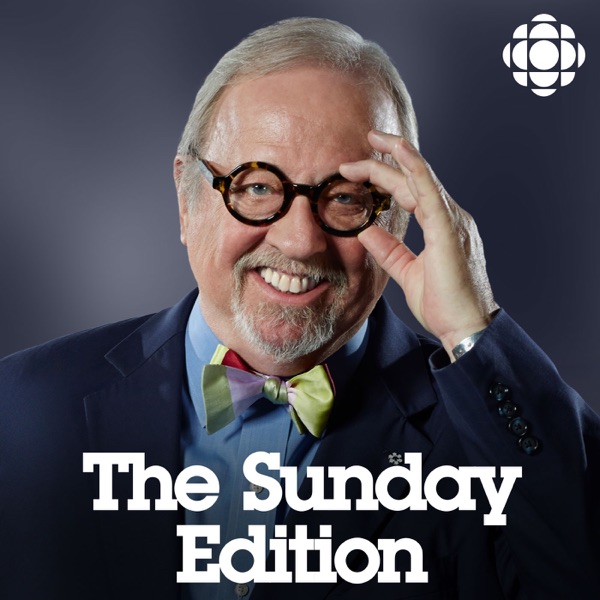The square-shaped image features an elderly man, likely in his 60s, centrally positioned and smiling warmly at the camera. His distinguishing features include a gray goatee, thinning hair, and round, turquoise glasses with a brown, multi-colored frame, which he is adjusting with his left hand. He is dressed in a navy blue suit jacket over a light blue shirt, complemented by a vibrant, multicolored bow tie in shades of green, red, yellow, and purple. The background is a dark gray, providing a stark contrast to his attire. At the bottom of the image, white text reads "The Sunday Edition," suggesting he is associated with a talk show or critique platform. In the upper right corner, a logo consisting of circular white symbols forms an overall round shape, presumably representing the publishing or production company. The image has a formal yet approachable feel, indicative of a promotional poster or advertisement.